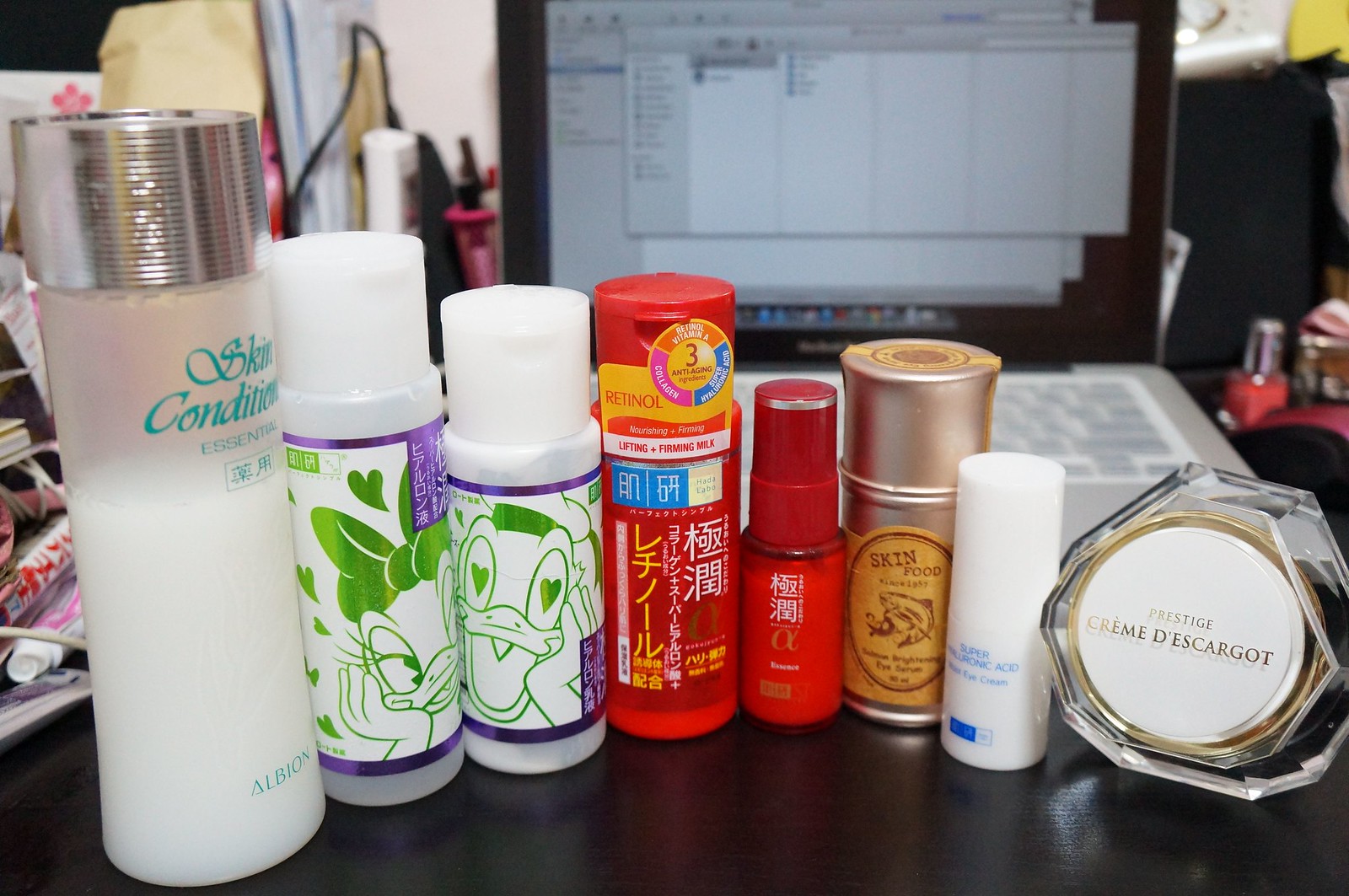This photograph features an assortment of Japanese skincare products meticulously arranged on a black tabletop, against a backdrop of a somewhat cluttered desk. In the background, a MacBook Pro displays an open File Explorer window, contributing to the chaotic scene alongside various beauty products and electronic devices.

The primary focus remains on the seven distinct skincare items arranged in a row. Starting from the left, the first product is a tall, clear container with a silver cap, filled with a white liquid. The label reads "Skin Conditioner," followed by the brand name "Albion" and some text in teal Japanese script.

Next to it is another tall, cylindrical bottle, this time opaque white with a holographic label featuring an image of Daisy Duck, along with Japanese writing and purple accents at the top and bottom.

Standing beside it is a smaller, similarly shaped bottle, distinguished by an image of Donald Duck on its front.

Continuing to the right, there is a slender red bottle bearing the label "Retinol 3," with additional Japanese text.

Adjacent to this is a smaller red spray bottle, also adorned with Japanese characters and white accents.

Following this is a silver metallic container labeled "Skin Food," decorated with a yellow and brown design.

Next is an even smaller, white cylindrical bottle, which appears to be labeled "Hyaluronic Acid" in blue text.

The final item is a unique, clear, gem-shaped container labeled "Prestige Crème d'Escargot," accented by a white label with a gold border, possibly made of acrylic.

The detailed variety and distinctive designs of these products highlight both the luxury and cultural aesthetics of Japanese skincare.